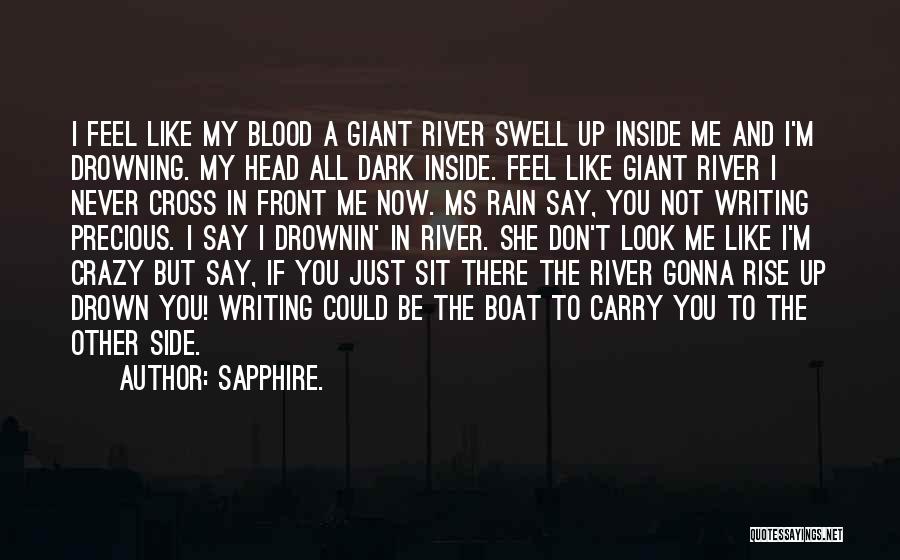This photograph captures an evocative quote overlaid on a semi-transparent, extremely dark background, hinting at a shadowy outdoor scene with barely discernible streetlights and possibly a skyline. The background may also suggest a sunset behind the darkness. The quote, written in centered white text, reads: "I feel like my blood, a giant river, swell up inside me, and I'm drowning. My head all dark inside. Feel like giant river, I never cross, in front of me now. Miss Rain say, you not writing precious. I say, I drowning in river. She don't look me like I'm crazy, but say, if you just sit there, the river gonna rise up, drown you. Writing could be the boat to carry you to the other side." The quote is attributed to the author Sapphire and is accompanied by the website "quotesayings.net" in the lower right corner.